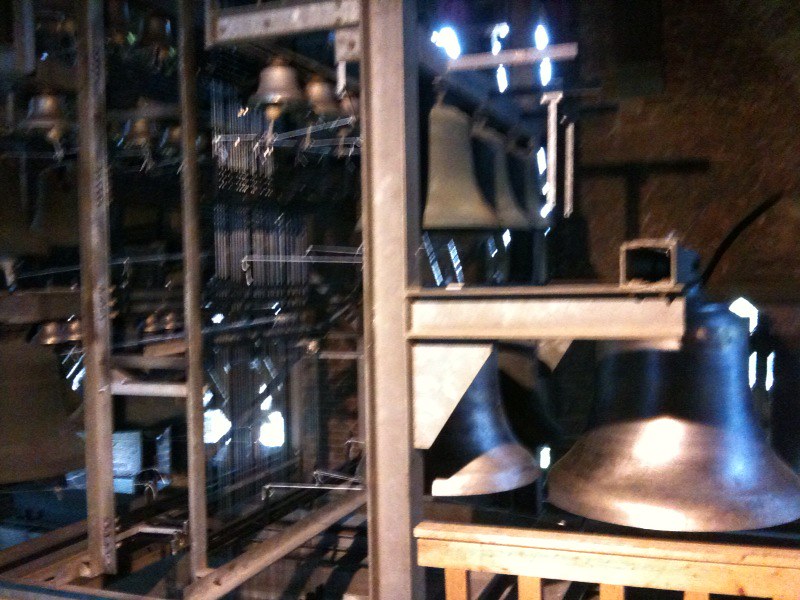The image depicts a large, dimly lit industrial warehouse or factory with a heavy emphasis on metal structures and components. In the center of the scene, there are approximately 30 sizable bells, reminiscent of those found in churches, suggesting that this location is dedicated to the production of such bells. The overall atmosphere is characterized by a dark, metallic tone, enhancing the industrial feel of the environment. Some sections of the photograph, especially towards the middle, are slightly blurred, potentially due to the motion of the person taking the picture.